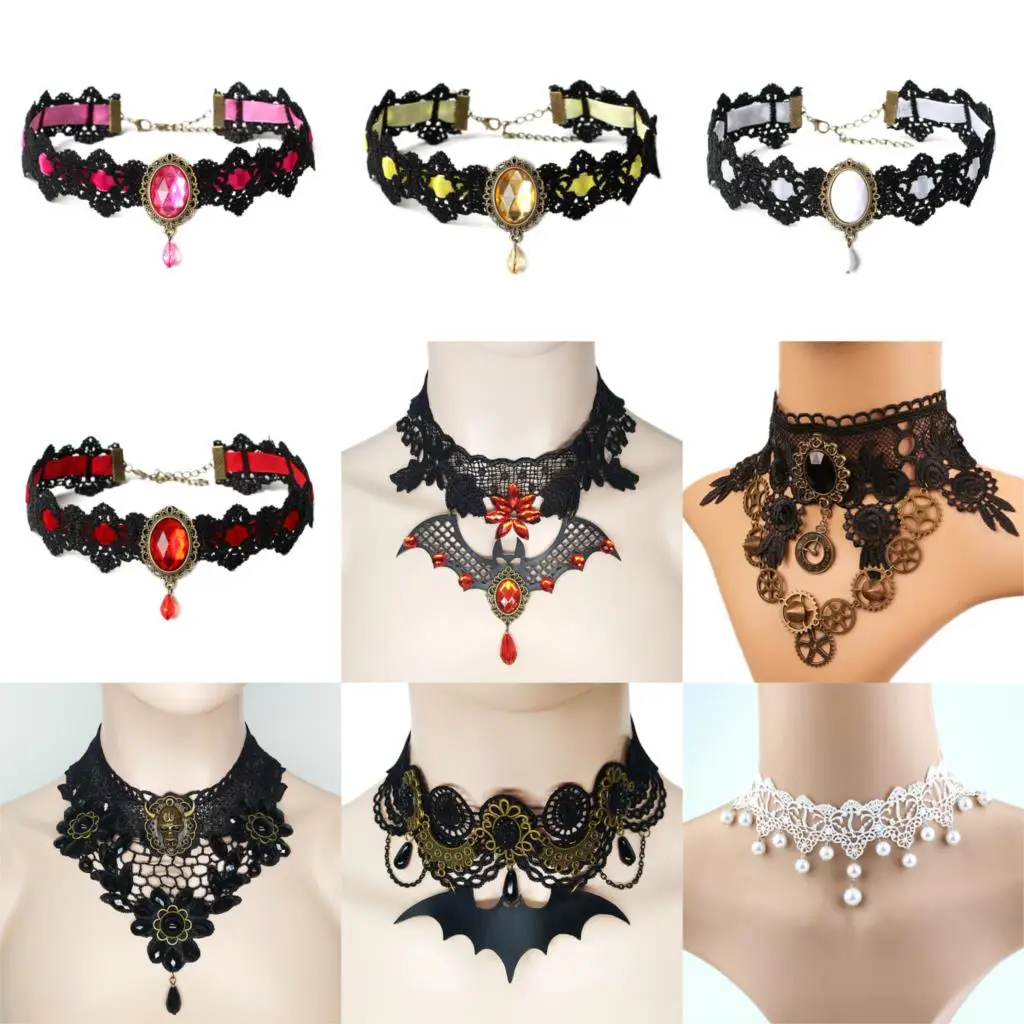The composite image displays a 3x3 grid of nine different necklace designs, each with a white background. The top row showcases three oval crystal pendants, bordered in gold, hanging from intricately designed black lace chokers. The necklaces differ by their primary colors: the left is pink, the middle is yellow, and the right is white. Each features a smaller crystal drop pendant beneath the main one. Directly below the pink choker in the second row is a similar necklace in red. Next to it, also in the second row, is a black lace choker adorned with a red flower and a metallic bat with hanging red jewels, and to its right, a black lace choker with dark gold and black gears. The bottom row continues with black lace necklaces: on the left, a choker embellished with floral patterns, and in the middle, a plain black lace choker with a bat. The final image on the bottom right displays a strikingly different design — an elegant white lace choker adorned with pearls, reminiscent of wedding jewelry.